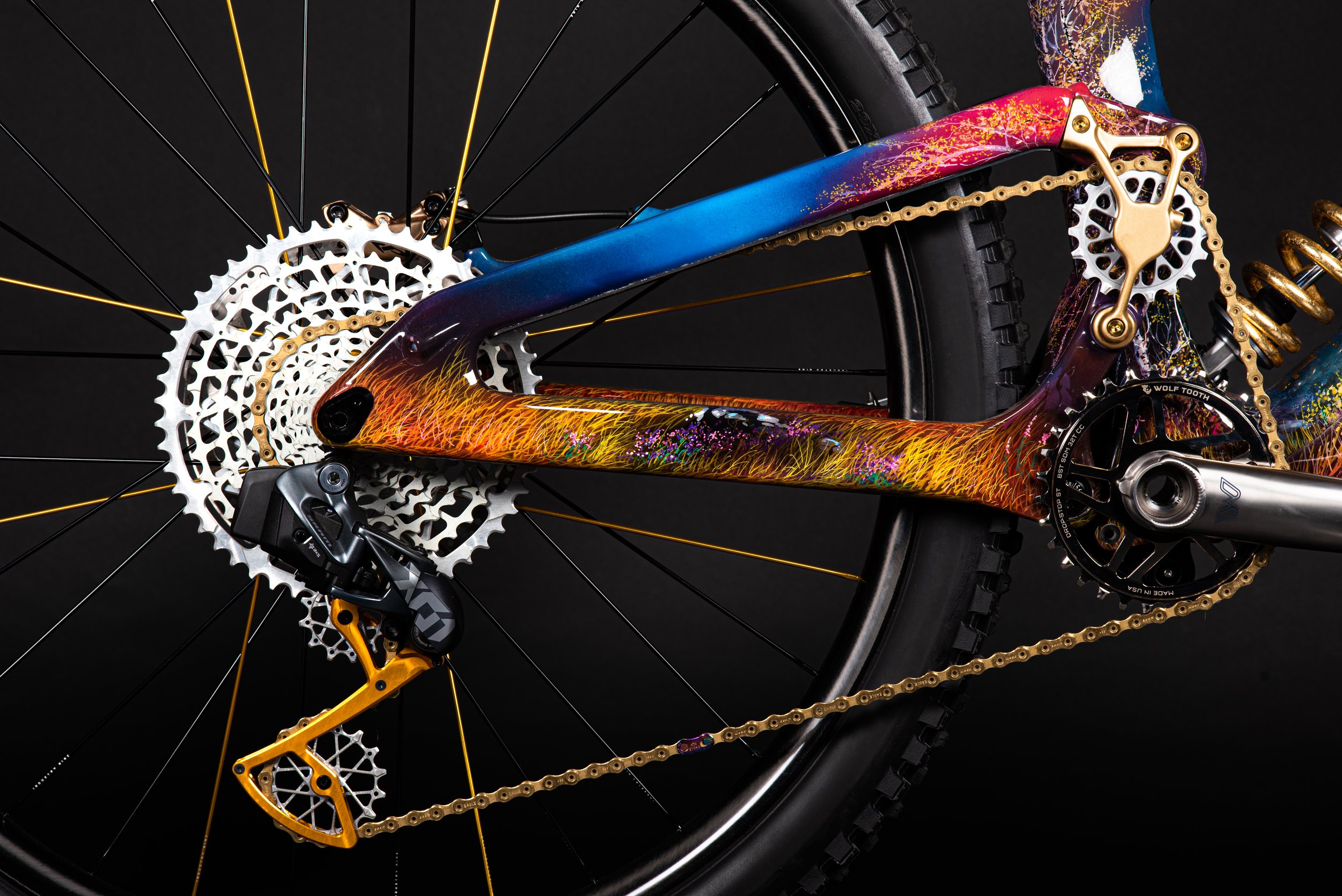The image captures a close-up view of the back wheel area of a multicolored bicycle, against a solid black background. The bicycle wheel itself is made of black rubber with visible tread, encased in a silverish carbon-colored rim. The spokes are thin, in varying hues of black, silver, and gold, emulating a visually striking effect. The central gear, as well as the bottom and front gears, are silver, surrounded by a golden chain that connects them. The bicycle frame stands out with an eye-catching paint job that gives an impression of paint drips or brush flicks, featuring predominantly purples, blues, and yellows, with the yellow paint appearing more flecked. Additionally, the frame includes touches of red, green, and a golden coil towards the right side. A silver bar or pedal cranks the gear, completing the bicycle’s colorful and artistic aesthetic.